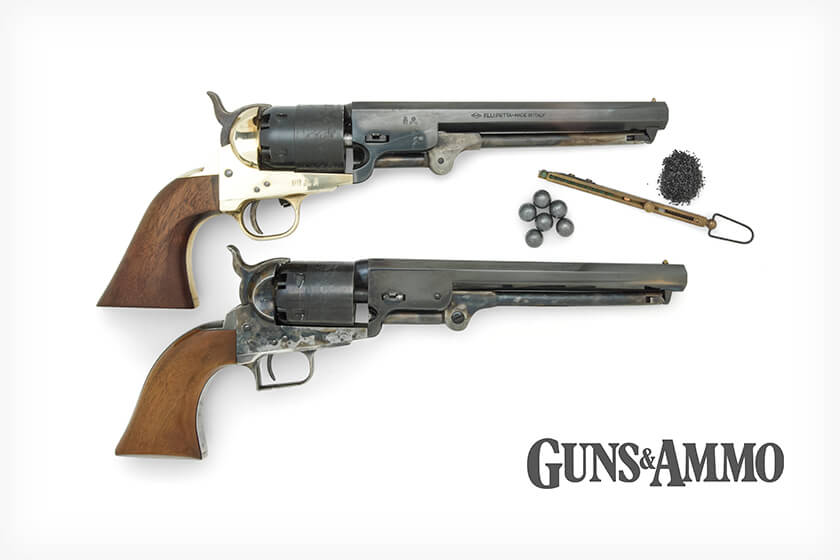This rectangular image, approximately six inches wide and four inches high, depicts two antique revolvers, reminiscent of those from the Wild West, laid side by side on a pale gray to darker gray gradient background. Both handguns, positioned horizontally with barrels pointing to the right and wooden hand grips to the left, feature a distinctive design that emphasizes their vintage appeal.

The upper revolver boasts a darker wooden handle and a dark gray, almost shiny metal barrel, with a near-ivory white coloration just above the trigger area adorned with what appear to be metal rivets. In contrast, the lower revolver has a lighter wooden handle and a more oxidized pewter-gray barrel, offering a slightly weathered look.

Nestled between the pistols is a small cluster of shiny gray lead balls, likely musket bullets, accompanied by a pile of fine dark gray gunpowder resembling tiny sprinkles. A slender metal rod with a ring on one end, possibly a tool for tamping down the gunpowder and loading the bullets, lies nearby.

In the bottom right corner, the text "Guns & Ammo" is prominently displayed in large gray print, completing the composition against the primarily white background.